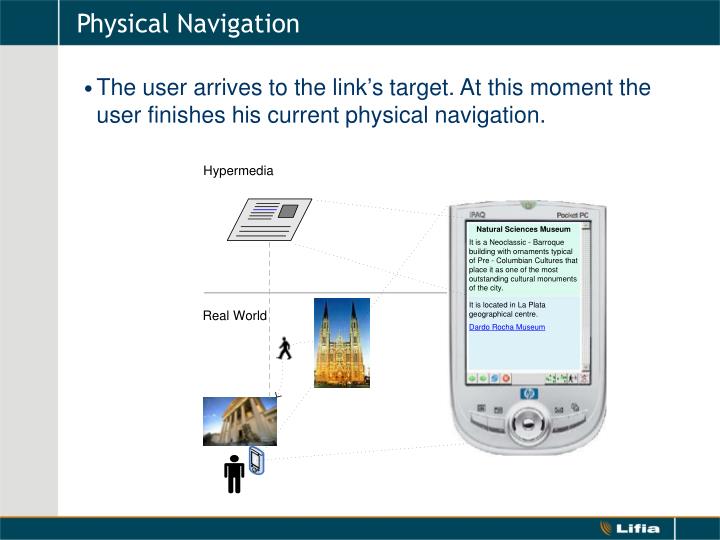The image is a presentation slide framed by horizontal dark turquoise, teal blue lines at the top and bottom. The top banner displays the title "Physical Navigation" in white text. Below this header, the main body of the slide has a white background. A prominent gray vertical bar runs along the left side. In the center of the slide, a teal-colored bullet point text states, "The user arrives at the link's target. At this moment, the user finishes his current physical navigation." To the right, beside this text, is an illustration of an old mobile device, possibly a pocket PC or a Blueberry phone, displaying the Natural Sciences Museum. The museum is described as a neoclassic Baroque building adorned with pre-Columbian cultural ornaments, marking it as a significant cultural monument in the city's geographical center, La Plata. Additionally, the slide includes the word "hypermedia" alongside an illustration of a postcard and the phrase "real world" paired with an image of a pedestrian and what appears to be a church. At the bottom of the slide, there's a dark teal banner with the word "Lithia" in white letters on the lower right side.